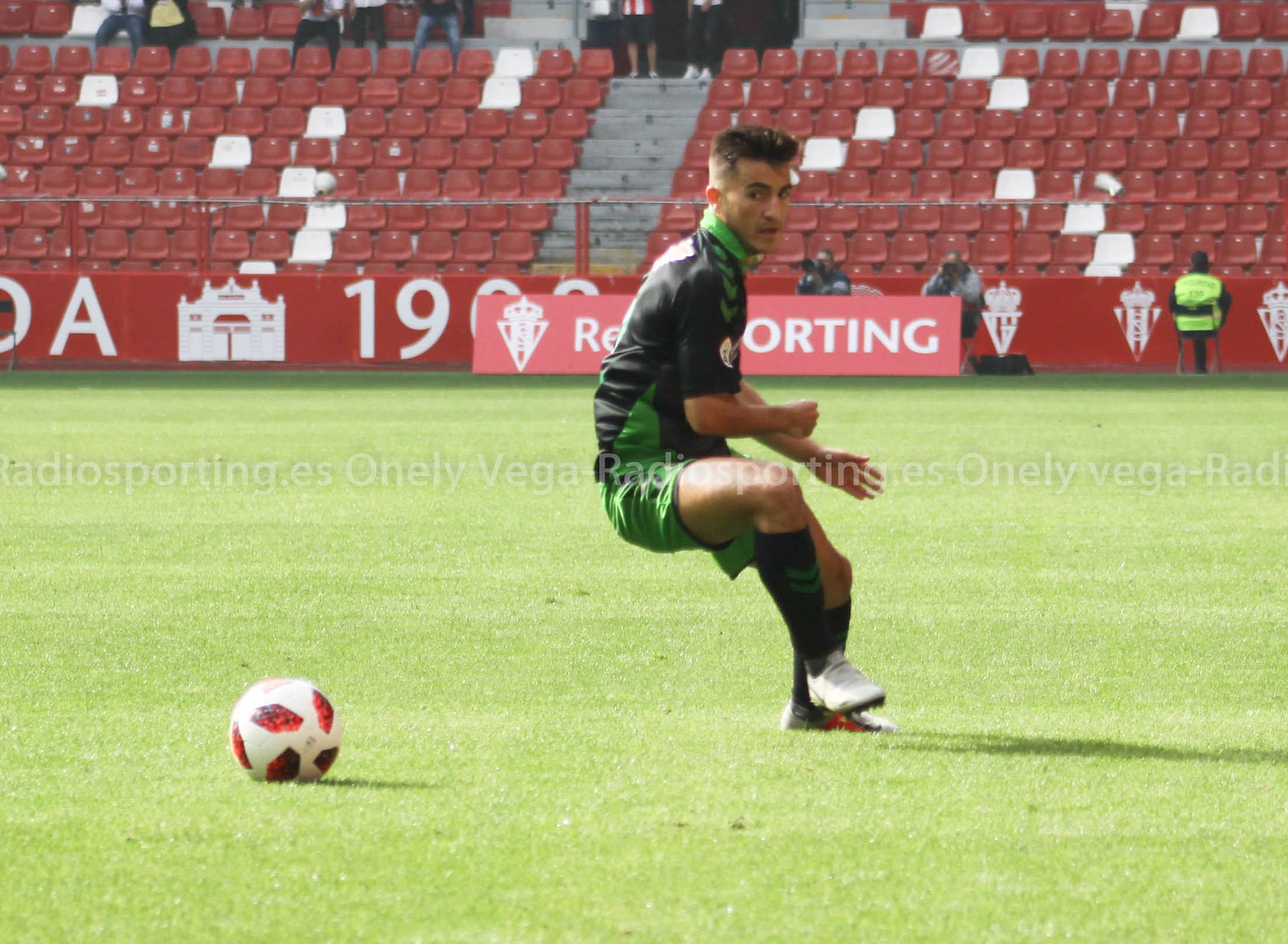In this dynamic image, a lone soccer player, mid-change of direction, is captured on an outdoor soccer field with vivid artificial grass. The player, sporting a black jersey with green accents on the sleeves and sides, green shorts with black stripes, and white soccer cleats, seems to be preparing for a swift turn as he glances over his shoulder towards a white soccer ball adorned with red spots. Black shin guards with green stripes complete his attire. The backdrop shows mostly empty stadium seats in red and white, with a few spectators and photographers standing on the sidelines, capturing the action. Prominently imposed across the center of the photograph is a white watermark reading "onelyvegaradiosporting.es," repeated in a banner-like fashion.